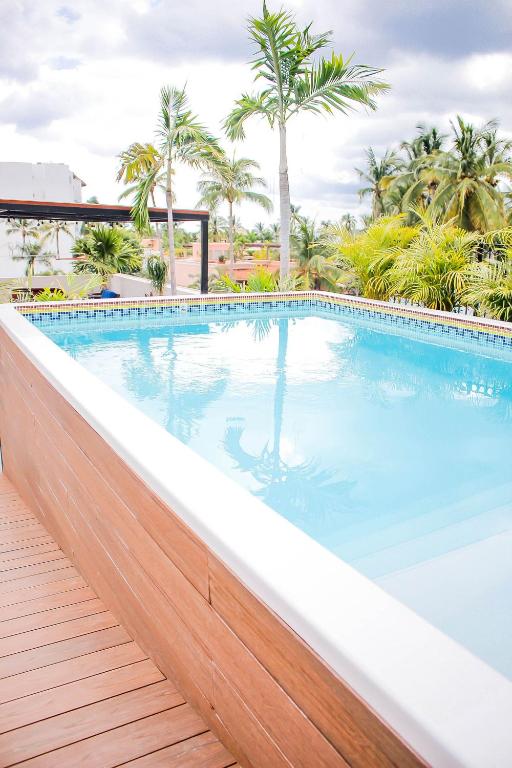The image showcases a picturesque, elevated pool framed by red wood panels and set on a dark brown or terracotta-colored wooden deck. The pool's water is crystal clear with a light blue hue, and there are steps visible inside, leading into the deeper end. Surrounding the top of the pool is an intricate tiled border featuring blue, yellow, and red designs. In the background, an assortment of palm trees with gray trunks and green and yellow fronds provide a tropical atmosphere. The sky above is a mix of dark blue and gray, indicating overcast conditions with prominent storm clouds. Notably, a pergola in a light natural wood color stands nearby, and in the far distance, a tall white building is visible. This setting gives off a relaxed, beach-like ambiance, reminiscent of locations such as California.